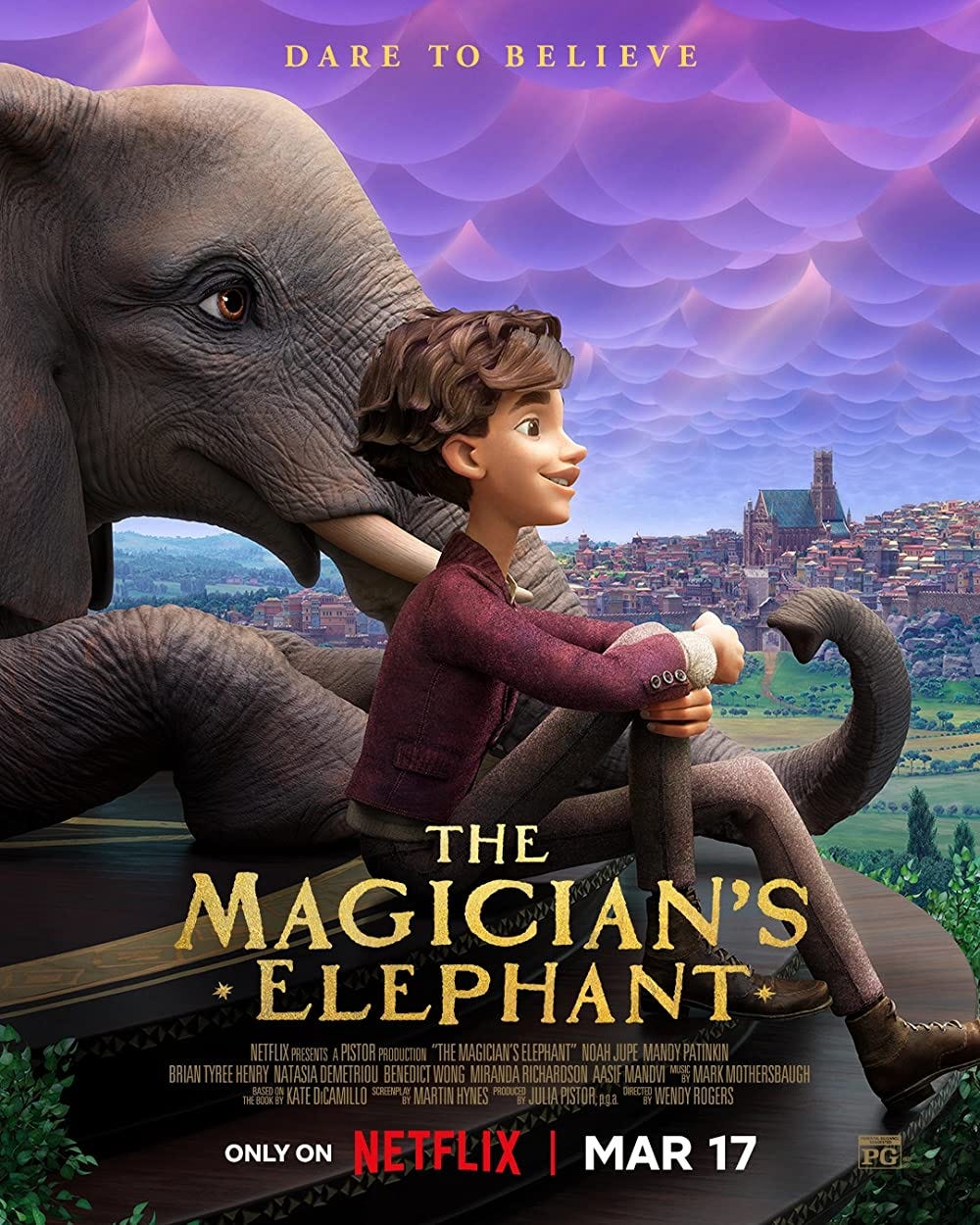The poster is an advertisement for a Netflix production titled "The Magician's Elephant," depicted in all caps gold font. Above the title, "Dare to Believe" is written in yellow letters. The poster features an illustration of a cartoonish gray elephant and a teenage boy with short, curly, fluffy brown hair, both gazing off to the right. Behind them stretches a field leading to a quaint town with red buildings, including a prominent church on a hillside. The sky above them is a striking purple color, adorned with whimsical, hanging, bubbly clouds. At the bottom, it states "Only on Netflix" in characteristic red font, accompanied by the release date "Mar 17" in white letters and the rating "PG." The poster includes cast names, such as Noah Jupe, Mandy Patinkin, and Brian Tyree Henry, and credits key contributors, including the book's author Kate DiCamillo, screenplay writer Martin Hines, and director Wendy Rogers.